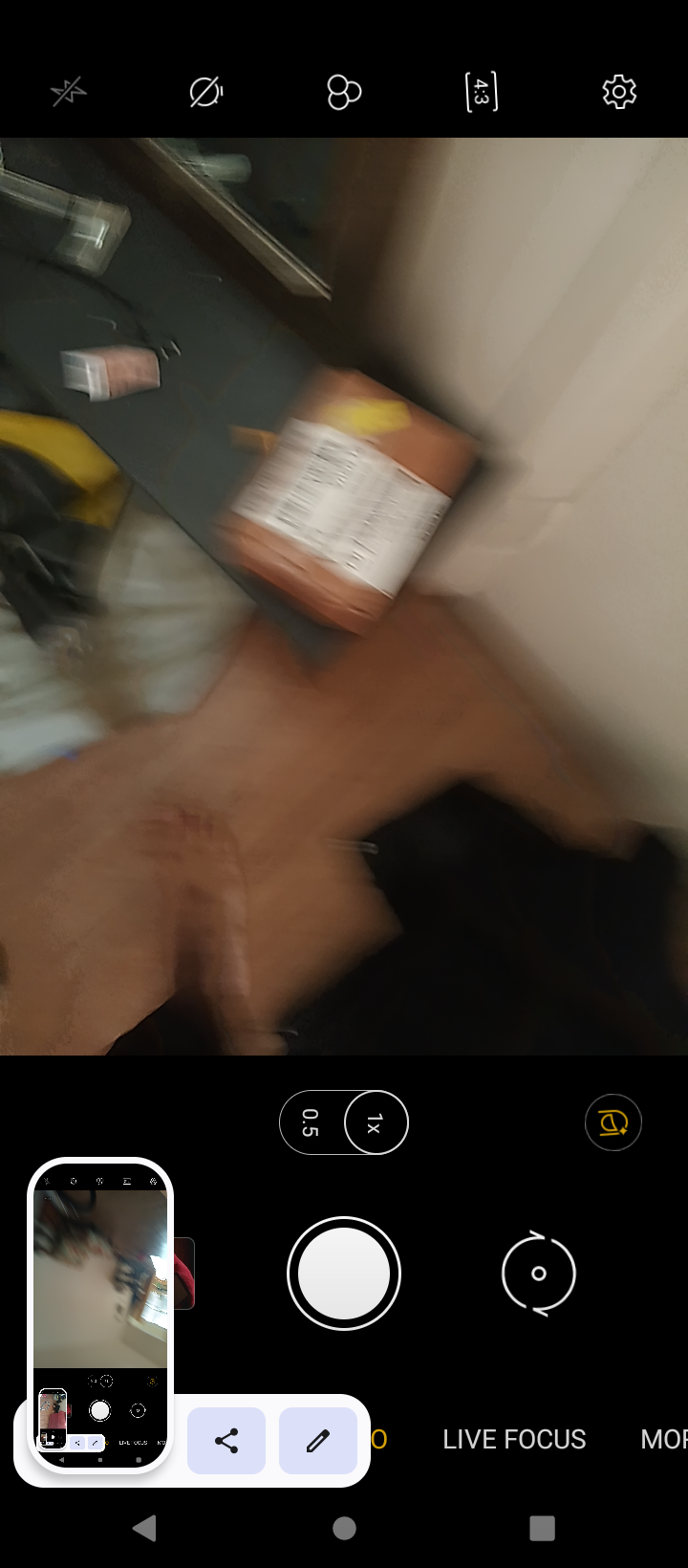The image is a color screenshot from a phone's camera app, captured in a moment of motion, making it quite blurry. The interface of the camera app is clearly visible, with the phone held sideways. You can see various on-screen elements including a gear icon for settings in the upper right, a 4:3 aspect ratio indicator, and other icons such as a set of three circles, a stopwatch with a slash, and a lightning bolt with a slash. At the bottom, there is a large circle for taking the picture, a flip icon with two arrows, a zoom indicator showing 1X within an oval that also displays 0.5, a gold-outlined person symbol, and partially obscured symbols including a pencil. 

The captured image depicts the inside of a room with several identifiable objects. Dominating the center is a rounded rectangular package, brown in color, with a white label that possibly contains black text and a barcode, situated on what appears to be a dark surface, possibly gray or green. There is a visible brown foot coming from the bottom left, adding to the casual and candid nature of the photo. The background includes a light brown hardwood floor, a white wall, part of a door, and a mirror. There's a black plug with two prongs and some black items, possibly furniture, in the bottom right. The curtains in the upper right are white. The entire composition suggests a domestic setting captured quickly and without proper focus, emphasizing the spontaneous nature of the shot.